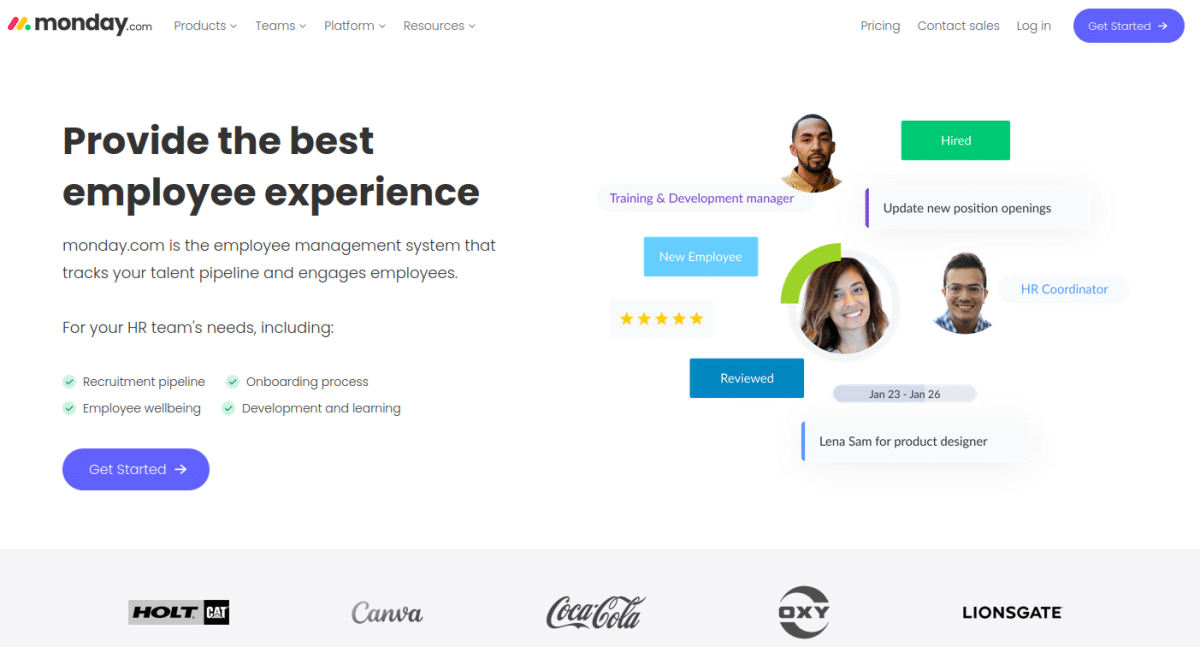**Screenshot Description: Monday.com Interface for Employee Management**

At the top left of the screenshot, there is a navigation menu featuring options such as: Monday.com, Products, Teams, Platform, Resources, Pricing, Contact Sales, Login, and Get Started. Below this, a tagline reads, "Provide the best employee experience. Monday.com is the employee management system that tracks your talent pipeline and engages employees. For your HR team's needs including recruitment pipeline, employee well-being, onboarding process, development and learning, get started."

To the right of this text is an image of a dark-skinned man, accompanied by the text "Hired. Training and Development Manager," indicating a new position opening. Nearby, there is a circular photo of a fair-skinned woman with long wavy hair, smiling warmly at the camera. Below, another image shows a man with glasses and short dark hair, also smiling at the camera. The text adjacent to his image reads: "HR Coordinator, reviewed Jan 23 through Jan 26, Lena Sam for Product Designer."

At the bottom, a gray border features the names of notable companies: Holt, Canva, Coca-Cola, Oxy, and Lionsgate, likely indicating partnerships or client endorsements. The overall image format is wider than it is tall, meticulously devoid of animals, plants, flowers, trees, or automobiles.